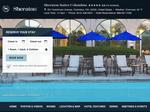A photograph is bordered at the top and bottom by black strips with white lettering, although the text is too blurry to decipher. The top left corner features a round symbol that is similarly obscured. The central part of the image showcases three pristine white archways, through which lush green trees are visible in the background. In the foreground, blue triangular shade covers are suspended, providing respite from the sun. Beneath these shade structures, verdant green bushes add a touch of natural beauty. To the right, a serene blue pool is encased by white concrete, and several white chairs are arranged neatly around it. On the left side of the scene, there is a white box that contains a blue section with black letters, though both elements are indistinct due to blurriness. The overall composition exudes a sense of calm and elegance, blending natural elements with structured architectural forms.